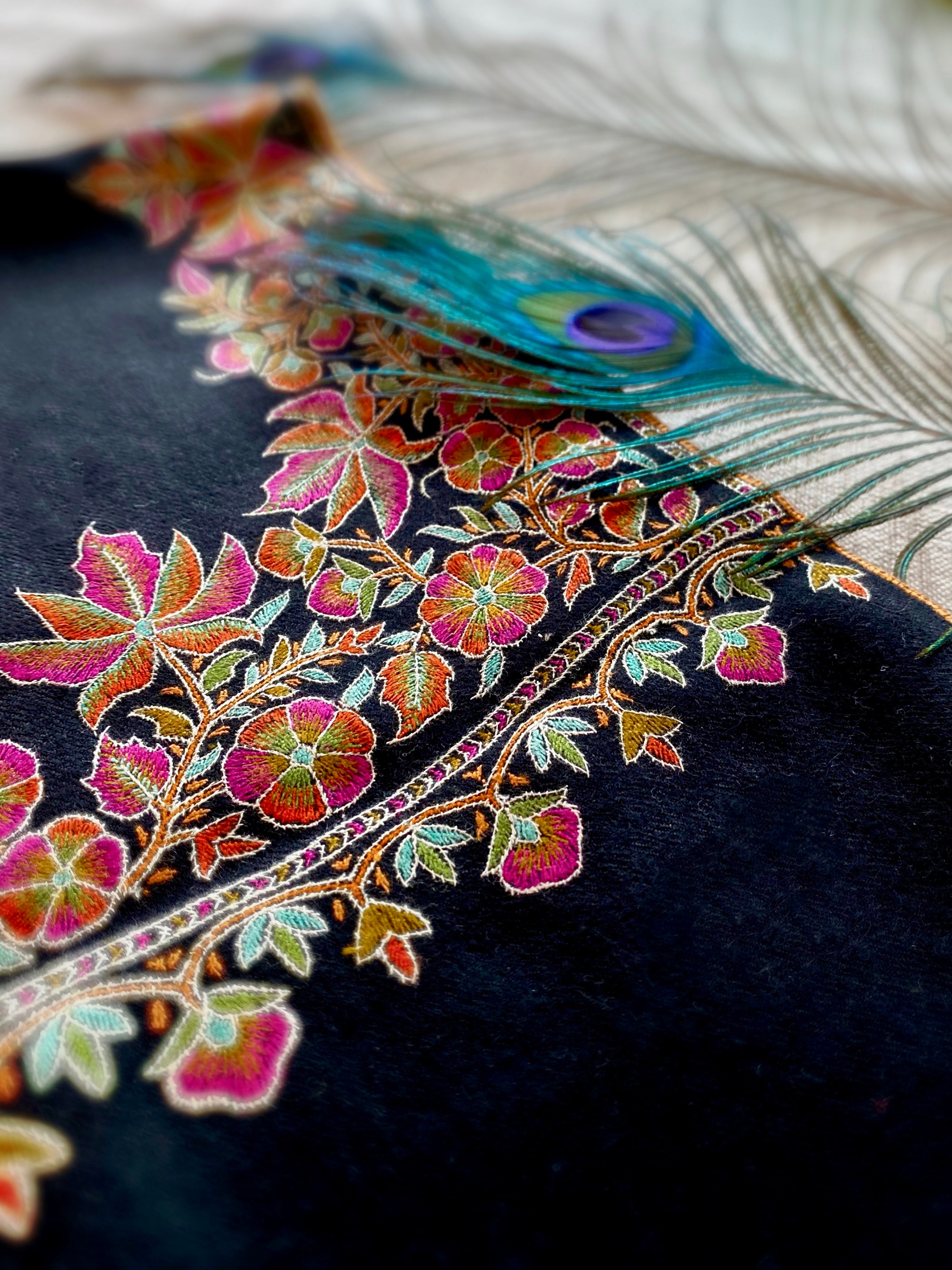This photograph showcases an intricately embroidered piece of cloth laid flat on a white background. The fabric itself is a deep navy blue, providing a striking contrast to the vibrant floral embroidery that adorns it. The floral pattern features an array of colors, including reds, yellows, pinks, oranges, and greens, intricately stitched to depict flowers and leaves. The embroidery extends across the cloth, reaching from the left side to the right and climbing up to the corner of the material. 

Amidst this detailed embroidery, a single peacock feather is prominently positioned, extending from the right side of the image. It boasts a spectrum of colors, from blue and green to a central purple circle with an inner black ring. The feather adds an elegant touch to the overall composition.

Surrounding the floral embroidery is a subtle gold border, further accentuating the detailed artwork. The cloth appears to rest on a white or beige surface, providing a calm and neutral backdrop that highlights the vivid colors and intricate designs of both the embroidery and the peacock feather, making them truly stand out.